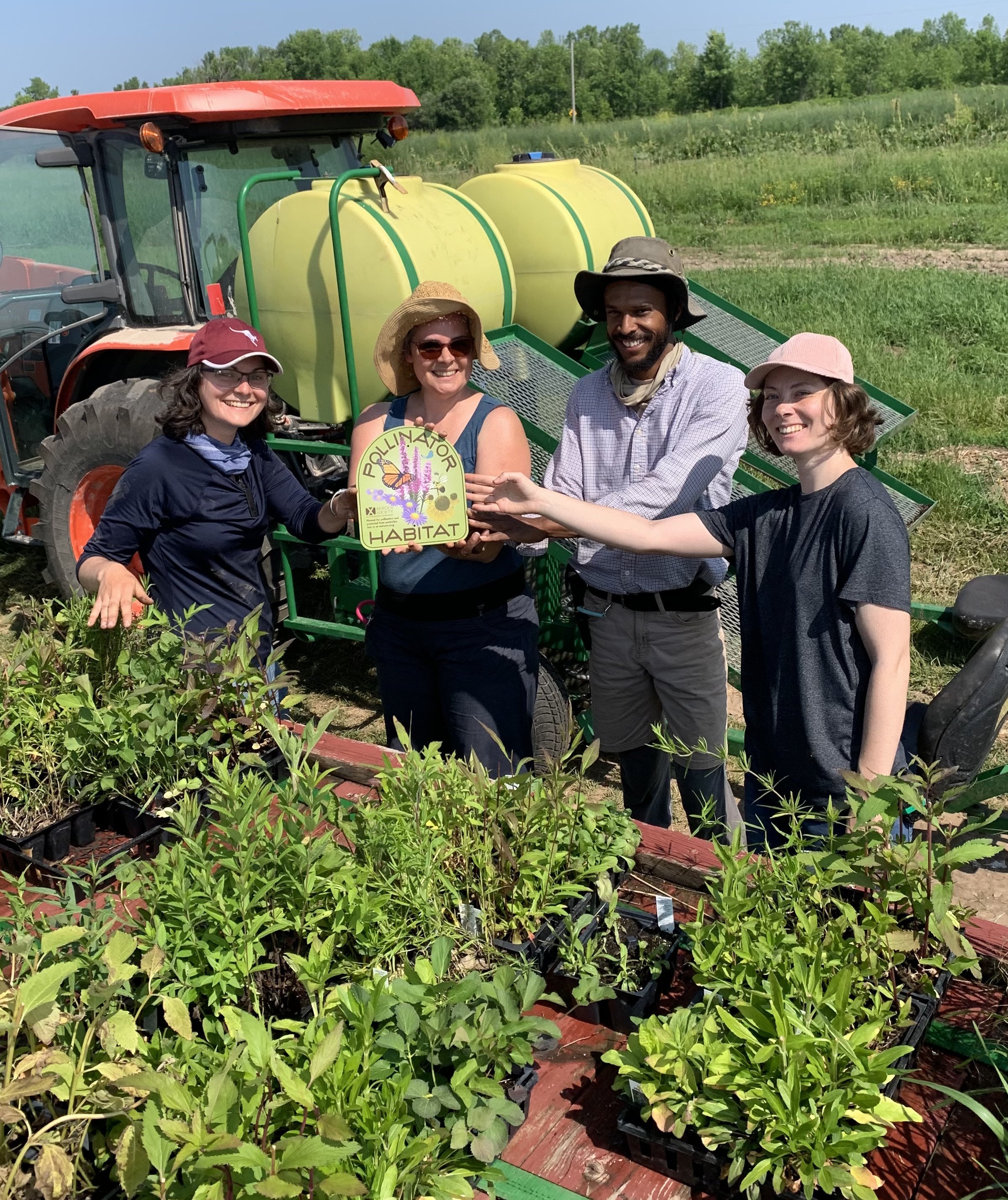In this detailed photograph set in a farming field during daylight, four individuals – three women and one man – are happily posing for the camera holding a sign that reads "Pollinator Habitat." The group is identifiable by their varied attire, suited for farm work, and distinctive accessories. Starting from the left, a Caucasian woman sports a long-sleeved navy blue shirt and a burgundy hat featuring a white kangaroo, while another Caucasian woman next to her wears a blue tank top and a light tan floppy hat. On the right side, another Caucasian woman with curly brown hair is seen in a long-sleeved black shirt and a pink baseball cap, and between her and the second woman, a black man is dressed in khaki pants, a light blue collared shirt, and a floppy gray hat.

They stand in front of a large red tractor equipped with a trailer carrying large yellow canisters with green stripes, likely used for distributing liquid or spray. Besides the tractor, the scene includes a reddish wooden wagon and an array of black planters housing green leafy plants, indicative of their farming activities and the "Pollinator Habitat" theme. In the background, the expansive green field and a distant tree line complete the picturesque agricultural setting.